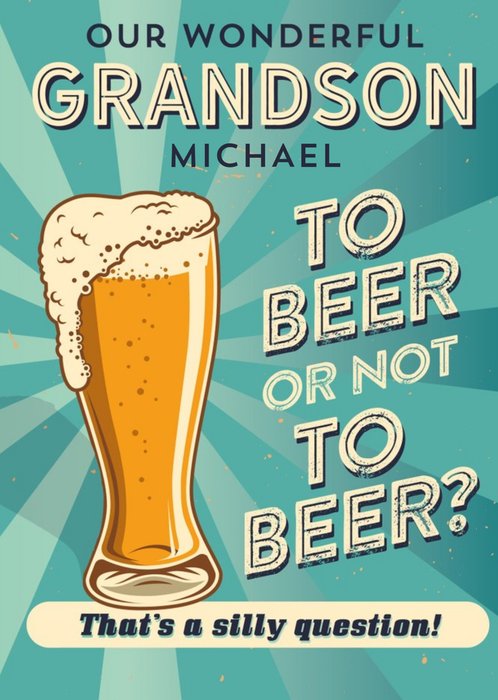The image is a vertically oriented, edited digital piece resembling a greeting card cover, blending digital art and text. On the left side, there is a detailed drawing of a beer glass filled with amber-colored liquid, topped with frothy white foam that drips down the left side of the glass. Emanating from behind the beer glass is a radiant striped pattern consisting of alternating light and dark blue shades, giving the impression of rays of light.

At the top of the image, in dark blue text, it says "R, wonderful," followed by "grandson" in larger, pseudo three-dimensional white text with a navy-blue outline. Below this, also centered, is the name "Michael" in smaller, navy text. Towards the right side of the image, the text "to beer" appears in the same large 3D style, followed by "or not" in the same style but not three-dimensional, culminating in the larger text question, "to beer?" In the banner-style cutout at the bottom of the image, which is white with rounded corners and spans from the right to the left side, stopping just short of the edges, it reads in navy text, "that's a silly question!"